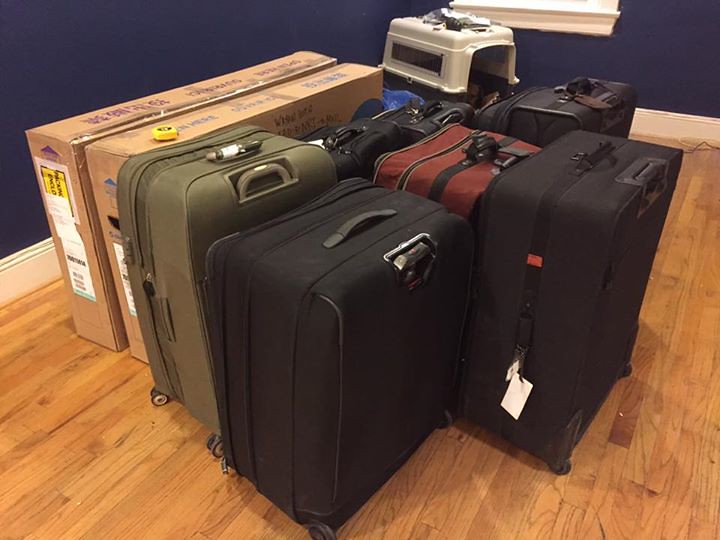The image displays an array of seven upright fabric suitcases, each equipped with wheels and handles, lined up in a neat arrangement on a pine wood floor. Five of the suitcases are black, one is red, and one is olive green with a military-like appearance. There are three larger suitcases among them. Situated to the left side are two large boxes that resemble TV packaging, and atop one box lies a yellow tape measure. In the background, there is a light gray pet crate, seemingly large enough for a dog as there's a faint outline of a dog's head visible through the crate's door. The room features dark navy blue walls with tall white crown molding, providing a striking contrast to the wooden floor. Some of the suitcases have visible tags, suggesting that their owner is preparing for travel, potentially to an airport.